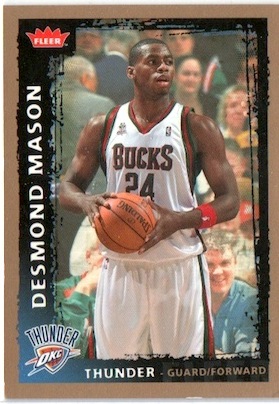This is a full-color sports trading card bordered in brown, with an inner border transitioning from black to blue. At the top, a red crown design prominently features the word "FLIR," indicating it is a FLIR card. The card showcases Desmond Mason, a muscular young black gentleman, who is identified as a guard/forward for the Oklahoma City Thunder (OKC). Mason is depicted wearing a Milwaukee Bucks jersey, number 24, in white with brown accents. He holds a basketball in front of him and gazes off-camera. In the background, a crowd with discernible faces, including a man in a blue shirt and another in a green jacket, appears to have been superimposed, resembling a television screenshot. Desmond Mason's name is displayed vertically on the left in white text against a black strip, with "Thunder" and "Guard/Forward" noted at the bottom.